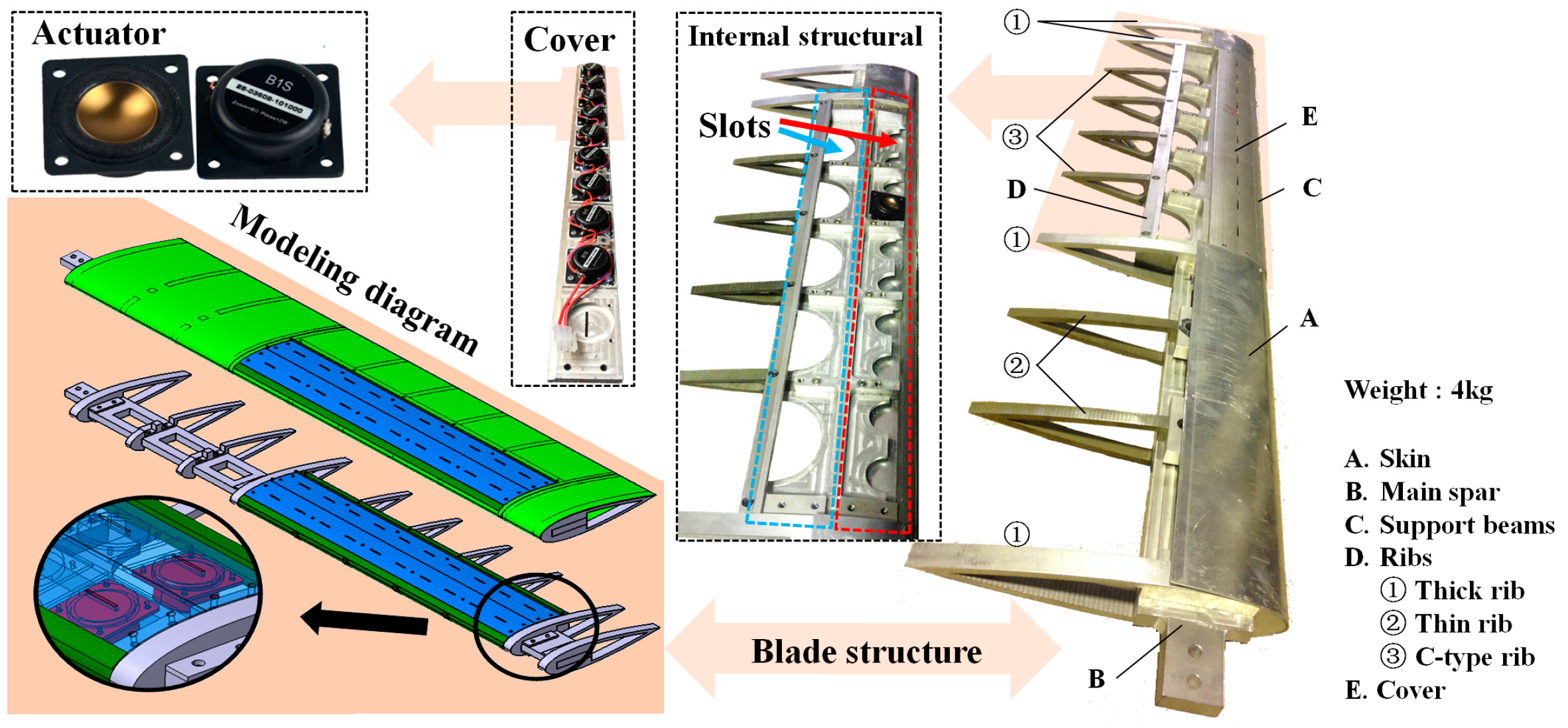The image depicts a detailed modeling diagram, likely of an aircraft wing, divided into several segments. In the top-left corner, there is an area labeled "actuator" with an illustration of an actuator device. Directly below, it states "modeling diagram," showcasing a partially green and blue wing structure with internal metal components. The visual highlights how the actuator integrates within this structure. Further annotations indicate sections titled "cover" and "internal structure slots," detailing various techniques and hardware elements associated with the wing.

Transitioning to the right section of the diagram, the anatomical breakdown of the wing continues, with labels corresponding to different parts: A for skin, B for main spar, C for support, D for ribs, and E for cover. Numerical labels identify specific types of ribs—1 for thick rib, 2 for thin rib, and 3 for C-type rib. The weight of the wing is noted as four kilograms, emphasizing the intricate engineering details.

Overall, the diagram comprehensively illustrates the structural components and assembly of the wing, providing insights into its design and functionality.